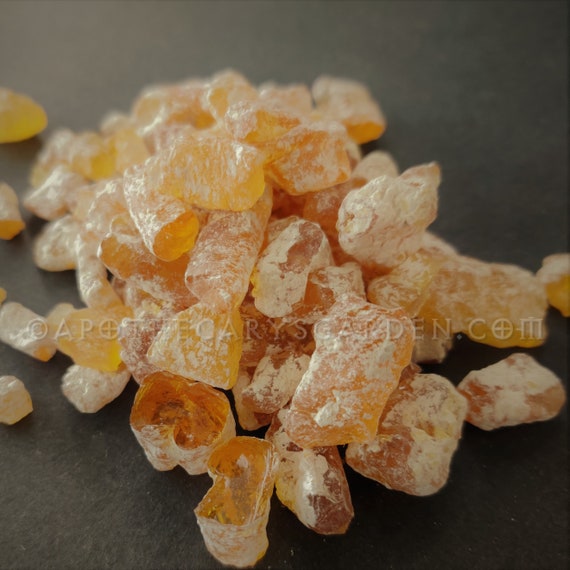The image showcases a close-up of numerous small, pebble-like nuggets scattered on a dark, black surface. These nuggets, numbering around 80 to 90, vary in shapes and sizes, and are coated with a white powdery substance. Some pebbles have been cut open, revealing their clear, amber to orange interiors reminiscent of a jelly or gel. The nuggets, possibly candies or dried fruit pieces, appear textured with a frosted layer on the outside. Prominently, the photograph features a watermark horizontally spanning across the image, reading "apothecariesgarden.com."